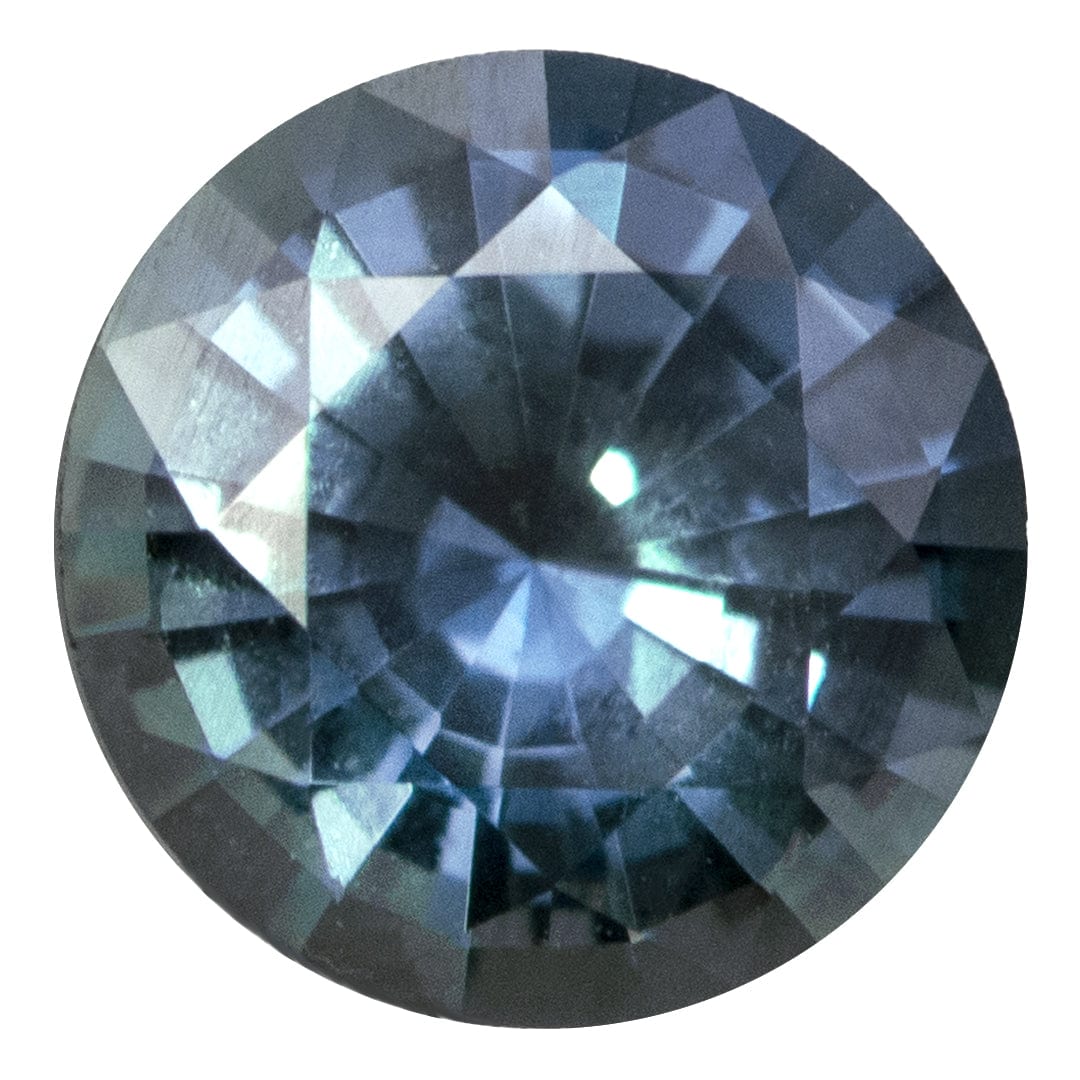This is an overhead view of a faceted gemstone, likely a dark blue sapphire. The stone is circular and exhibits a complex pattern made up of overlapping triangular facets, creating an intricate geometric design. Different shades of purple and blue, interspersed with flecks of white, enhance its visual allure and give it a sparkling effect. At the center of the gemstone, a subtle square shape is noticeable, accentuated by the interplay of light and shadows among the facets. The overall design also creates an illusion of narrow triangles converging toward the middle. The gemstone is not set in any setting and is displayed against a white background, emphasizing its vivid colors and intricate details.